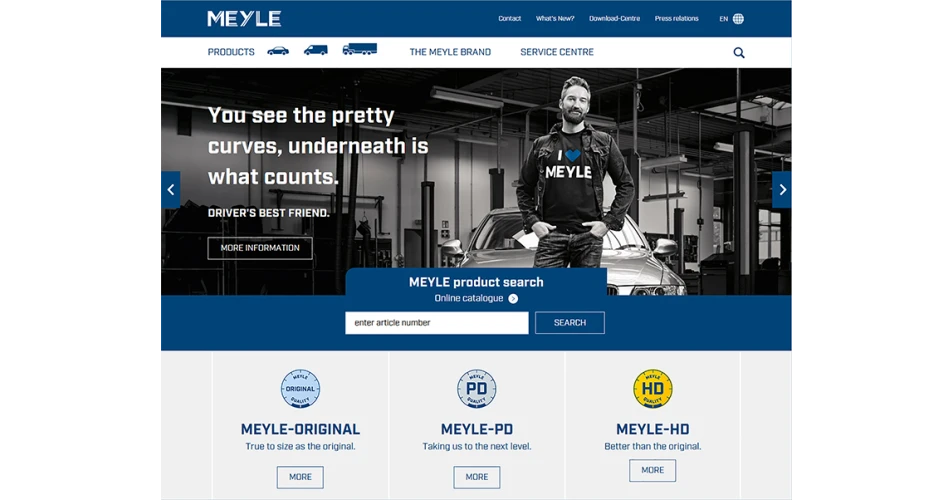**Detailed Caption for the Image on the Company Website:**

The top banner of the company website is a solid blue with the name "MEYLE" prominently displayed on the left in bold white font. On the right side of the banner, there are small, almost indiscernible letters ending in "EN". Also visible is a round emblem with an X-shaped design inside it. Just below this banner, there is a white section with blue text that reads "Products," featuring icons of a car, van, and a large truck. Adjacent to this, the terms "The MEYLE Brand," "Service Center," and a magnifying glass icon for a search function are displayed.

Directly below this, on the left, white text reads, "You see the pretty curves underneath is what counts," next to a blue box with a leftward-pointing white arrow. Underneath this phrase, a smaller white box contains the text "Driver's best friend" next to another box with "More information" written inside it.

In the main image area, a man with short hair and a beard stands on the right side, dressed in a black t-shirt that says "I love MEYLE" with a blue heart symbol. Behind him, a gray car is parked against a backdrop of gray walls and a black ceiling adorned with hanging light fixtures.

To the right of this image, a gray box with a white leftward-pointing arrow features prominently. Below this is another gray box with the text "MEYLE Product Search" in white font. Beneath this, the words "Online Catalog" are displayed with a white circle icon next to a white box that prompts users to "Enter article number" in gray font. A blue square with white font reads "Search". Below the gray section, a blue circle with the word "Original" in it appears, followed by the phrase "MEYLE Original, true to size as the original" in blue lettering.

Below this, separated by a white spacer line, there is another gray box and circle marked "PD". In blue font, it reads "MEYLE-PD" with the tagline "Taking us to the next level" beneath it. Another gray square labeled "More" is also present.

Further down, another white spacer line separates the next section where a yellow circle with the letters "HD" appears. Below this, the text "MEYLE-HD" is displayed in blue font, followed by the phrase "Better than the original". Below this, a blue square with the word "More" is visible. Finally, the description notes the presence of another gray box in the layout.